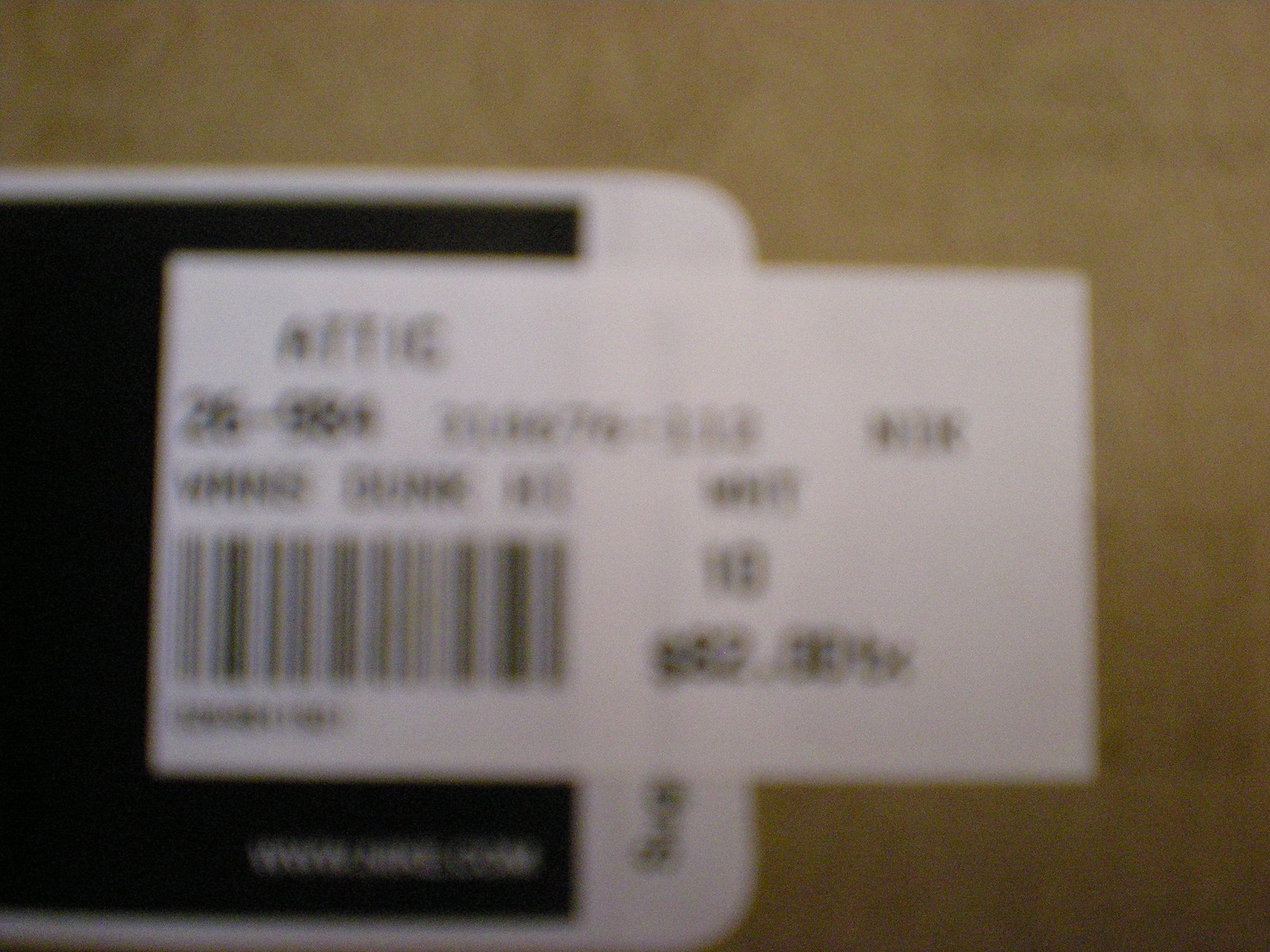This is an extremely blurry digital photo taken indoors. The background features a dark cream or light brown carpet visible in the upper left, upper right, bottom right, and center. At the heart of the image lies an item with a partially visible barcode tag. A white rectangle, presumably the tag, extends off a set item, draping over a smartphone. The smartphone, predominantly out of frame on the left, has white edges and a black screen. Within the white rectangle of the tag is a black rectangle; the bottom right corner reads "nike.com" in barely discernible white text. The black rectangle is flanked by another white section containing black text and a barcode, though the text is unreadable due to the extreme blurriness of the image.